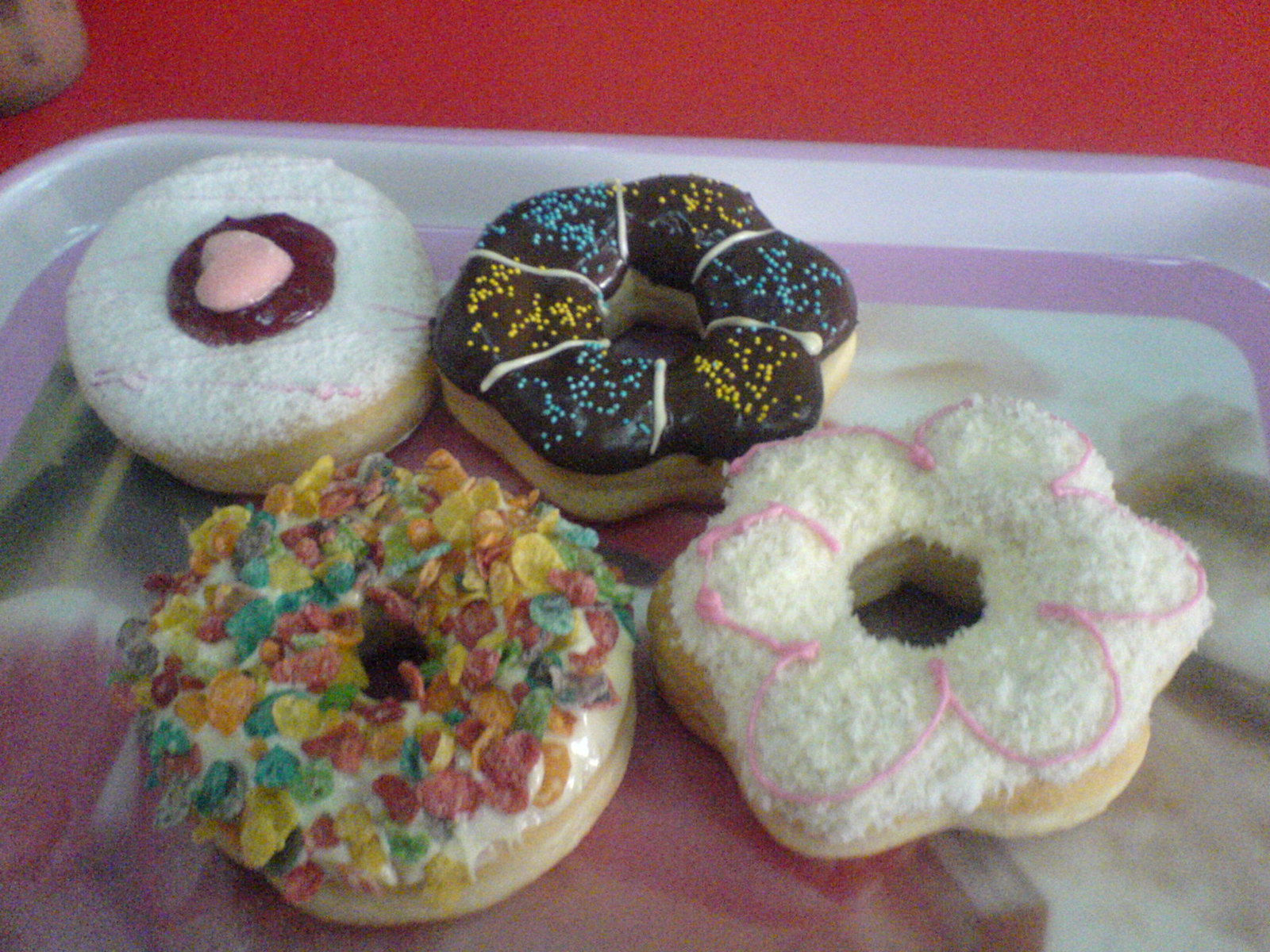This image features an overhead, front-facing view of four distinct doughnuts neatly arranged in a two-by-two layout on a shallow white and pink tray with a floral design and a purple lining on the edge. The tray rests on a red surface, with a small brown object, possibly a cup, visible in the upper left corner.

1. **Top Left Doughnut**: A circular doughnut with white frosting, adorned with a red jam circle in the center, and a pink heart at its core.
2. **Top Right Doughnut**: A hexagonal, flower-shaped doughnut with a light brown base, covered in chocolate frosting. This doughnut has white lines creating sections filled alternately with blue and yellow sprinkles.
3. **Bottom Left Doughnut**: A ring-shaped doughnut coated in white frosting and generously topped with colorful Fruity Pebbles cereal pieces in hues of red, orange, yellow, and blue.
4. **Bottom Right Doughnut**: Another flower-shaped doughnut with a light brown base. It has a white, textured, coconut-like frosting and is outlined with a delicate pink icing, mimicking the shape of a flower.

The tray’s intricate design and the vivid colors of the doughnuts create a striking visual contrast against the red background.